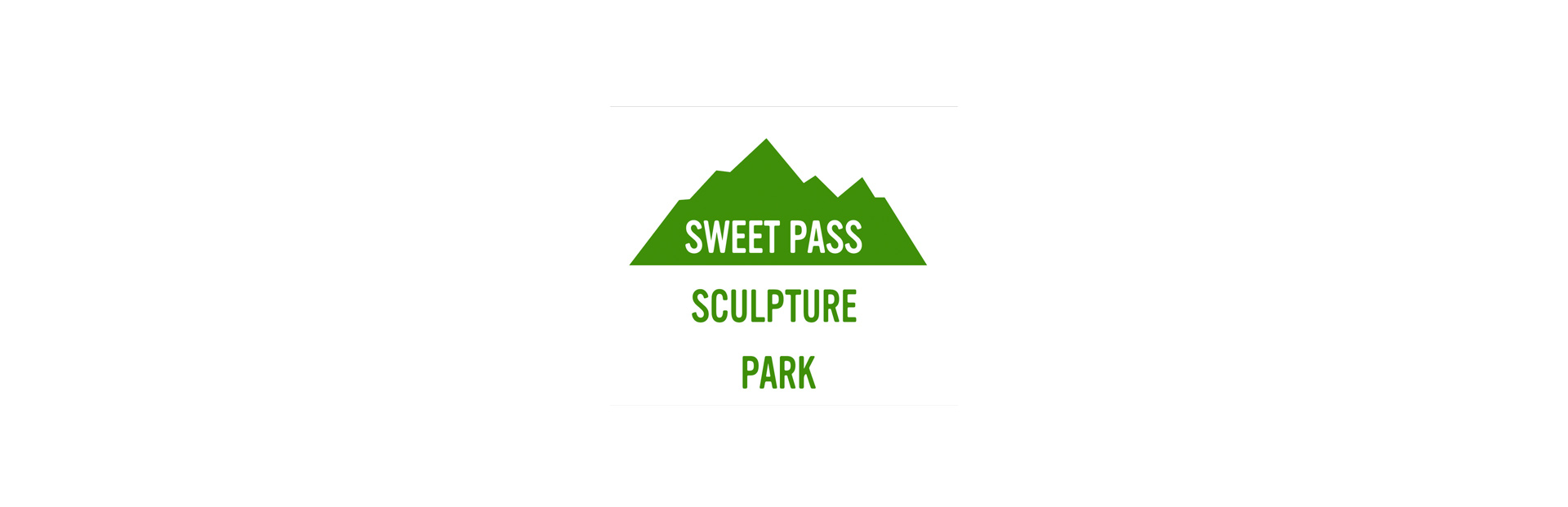The image features a small, contemporary sign with a plain, white background. At the center of the sign is a bright evergreen green graphic, depicting a stylized mountain range with sharp, triangular ridges. Positioned within this green mountain silhouette are the words "Sweet Pass" written in crisp white font. Beneath this graphic, in the same shade of green as the mountain silhouette, the text reads "Sculpture Park." The sign utilizes only two colors—white and green—creating a simple yet eye-catching design that clearly communicates the park's name and suggests a mountainous nature. The clean, minimalist design with the uniform font adds to its modern aesthetic.